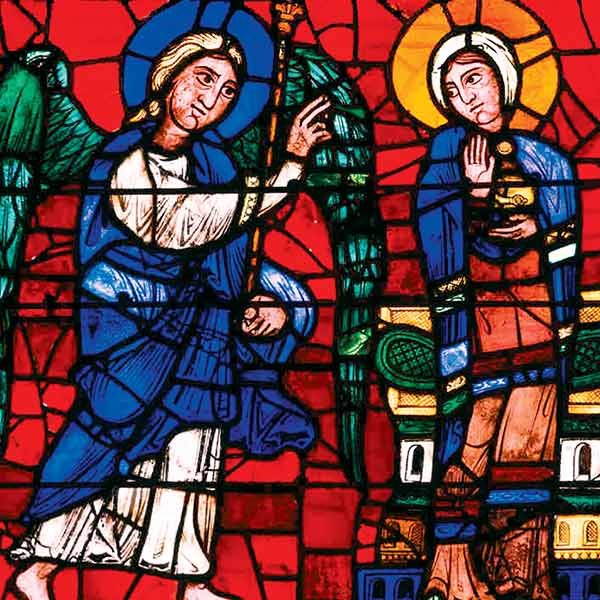The image showcases a detailed stained glass window featuring two central figures, possibly depicting a religious scene with the Virgin Mary and an angel. The woman, who could be the Virgin Mary, is depicted with a yellow halo around her head, dressed in a blue cape over her shoulders. She is holding a golden object close to her chest with her left hand and raising her right hand in a wave. The man beside her, identifiable by his green angel wings and a blue halo, is a white man with blonde hair. He is wearing a blue cape over a white robe and is holding a scepter in his left hand, while his right hand is raised toward the woman. The intricate background of the stained glass window features vibrant red panels with green and gold elements, possibly representing a building or a chair behind the woman. The overall scene is rich with religious symbolism and vivid colors, creating a striking visual narrative.